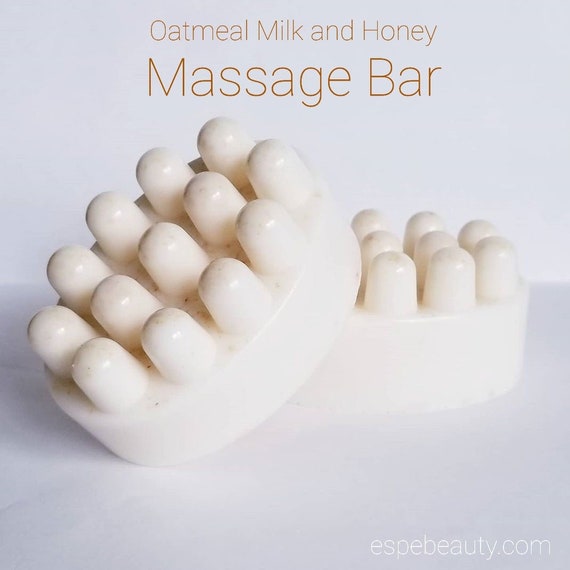The advertisement features two bars of soap against a light gray, nearly white background. One bar is lying flat, while the other is propped diagonally against it. These white, creamy bars are textured with small nubs intended for massaging during use. The nubs are roundish, with approximately 13 to 15 on each bar. Above the soap bars, text in a light brown or orangey-brown color reads "Oatmeal Milk and Honey Massage Bar." At the bottom right corner of the image, the website "spbeauty.com" is displayed in white lettering. The photograph is realistic, showcasing both the product and its intended use in detail.